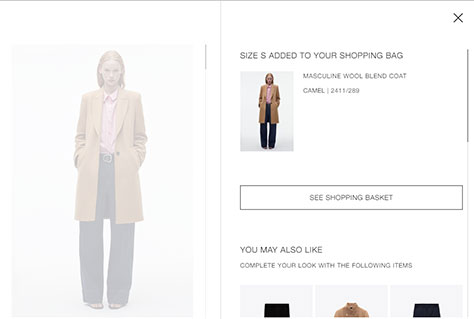The image appears to be a screenshot from an online shopping website. At the very top of the screen, there is a solid black bar. Below it, the page is divided, with a slightly hazy image on the left and a clearer screen on the right.

On the left side, there is an image of a woman wearing a long brown coat that extends almost to her knees. She is dressed in dark pants and a pink shirt and appears to have blonde hair. This image has a slightly hazy quality to it.

To the right, at the top, there is an 'X' in the upper-right corner, followed by the text "Size Small added to your shopping bag". Beneath this, there is a clear rectangular section displaying the same image of the woman in the brown coat. Beside this image, the text reads "Masculine Wool Blend Coat, Color: Camel."

Below this section, there is a button labeled "See Shopping Basket." 

Further down, the text "You may also like" appears, followed by the suggestion to "Complete your look with the following items." Underneath, three partially visible squares present additional items. The first square, with a grayish background, appears predominantly black. The second square shows a portion of a brown article of clothing, and the third square reveals another black item.

This detailed layout provides a clear snapshot of the online shopping experience depicted in the image.